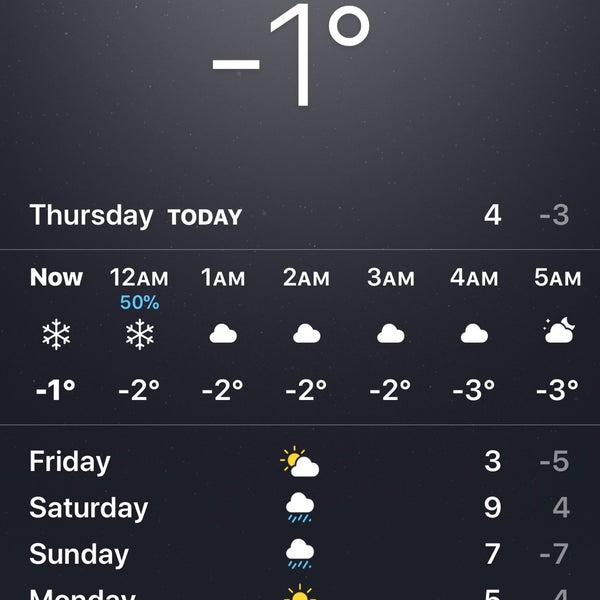A detailed screenshot from a weather application displays current and upcoming weather conditions. It shows that the present temperature is -1°, though the unit (Celsius or Fahrenheit) is not specified. The date reads as Thursday, the 4th of the month. The current weather condition is snowy with a temperature of -1°C. The temperature is projected to remain at -2°C with a 50% chance of snow at 12 a.m., and will stay at -2°C until 4 a.m. when it drops to -3°C. At 5 a.m., the temperature remains at -3°C.

Forecasts for the following days include:
- **Friday:** A high of 3°C and a low of -5°C, with some sun expected.
- **Saturday:** Rain is predicted with a high of 9°C and a low of 4°C.
- **Sunday:** More rain anticipated, with a high of 7°C and a low of -7°C.
- **Monday:** Partially visible, indicates sunshine with a high temperature of 5°C and a low of 4°C.